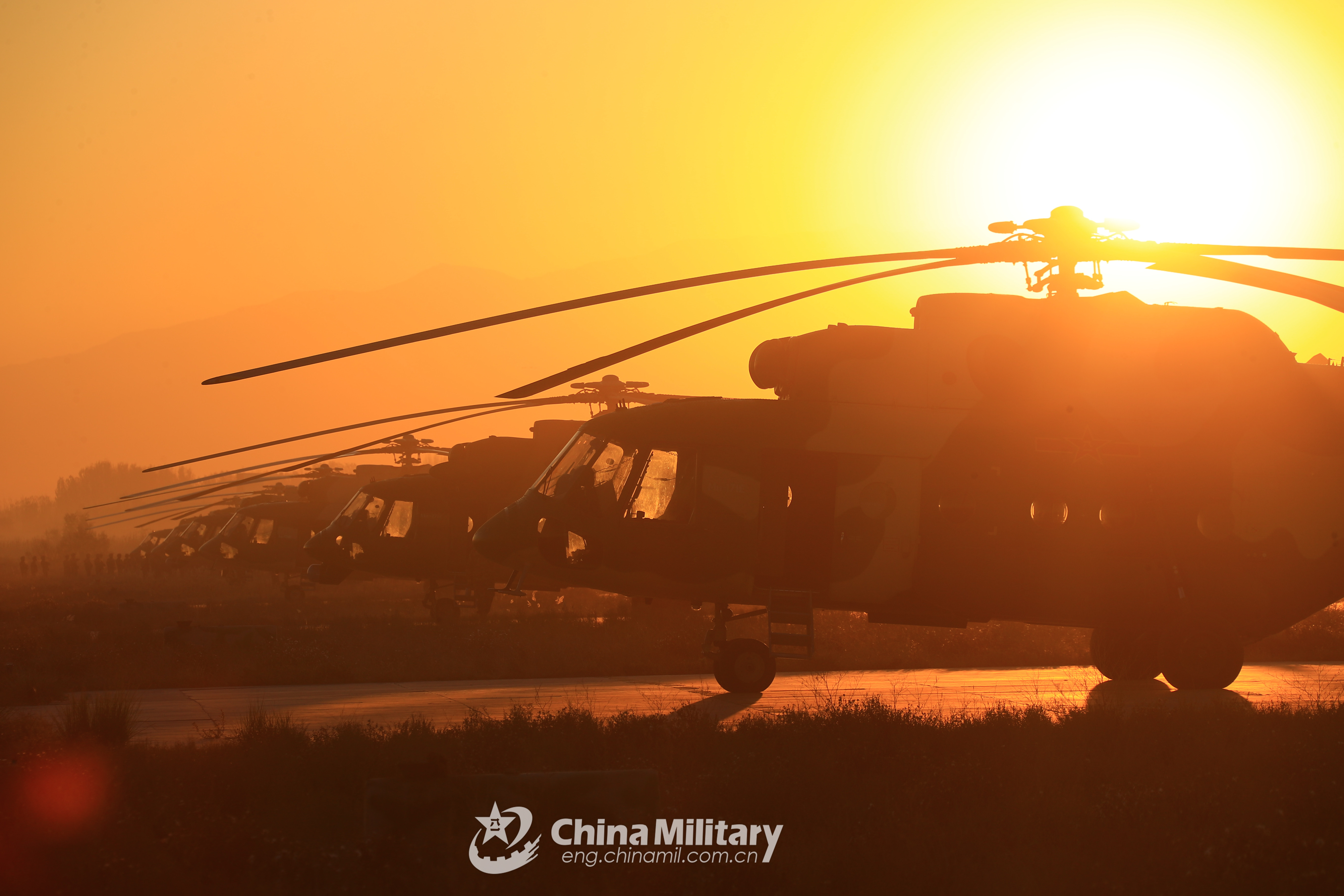This image, likely an action-packed military scene from China, showcases a row of five large helicopters with wide, glass-fronted cockpits. The aircraft are aligned on a paved surface, slightly offset from each other, creating a dynamic composition. The helicopters are parked, with a single front wheel and two larger rear wheels visible. 

Beyond the helicopters, the landscape features silhouetted grass and a distant row of trees, adding depth to the scene. The sky dominates the upper half of the image, painted in striking hues of orange, red, and yellow, intensifying the sense of a sunset shrouded in a dusty haze. A bright, bursting sun is positioned in the top right corner.

Near the horizon on the left side, a line of small, silhouetted soldiers is visible, adding a subtle human element to the vast scene. White text at the bottom of the image reads "China Military," with a smaller line underneath that says "eng.chinamil.com.cn." To the left of this text, there is a logo featuring a white star with a Chinese character, accompanied by a crescent moon and an arc or "swoosh" symbol beneath them, all contributing to the official and striking nature of the photograph.